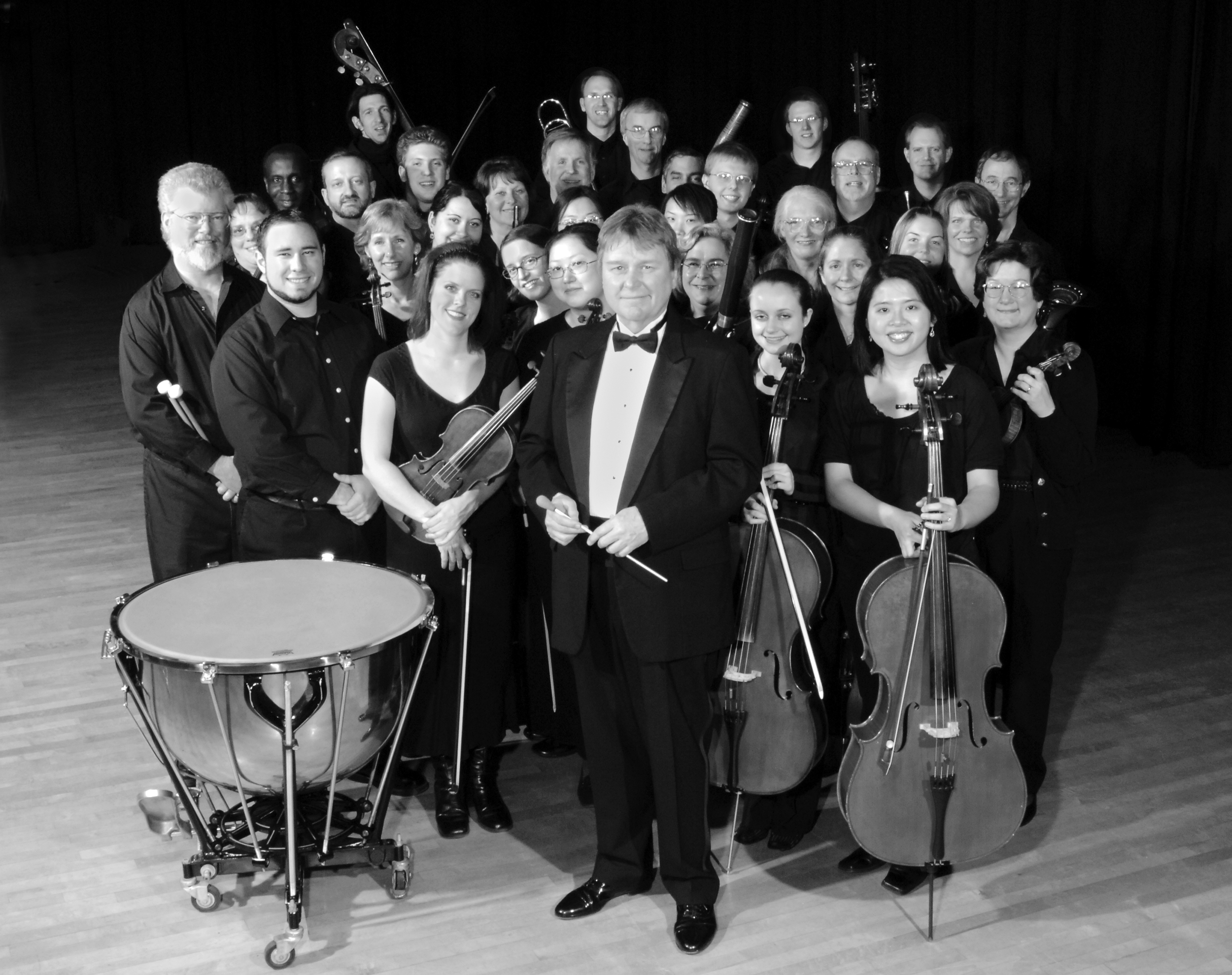This black-and-white photograph, approximately six inches wide by five inches tall, captures an indoor scene of a large orchestra ensemble taken from a slight elevation, providing a vantage point that looks down on the group. At the center of the image stands the conductor, a Caucasian man dressed in a tuxedo with a black bow tie, holding a baton in his hands. He is surrounded by 20 to 30 musicians, all standing together in a tight formation, smiling at the camera. To his right, two women hold cellos, while to his left, a woman holds a violin. Additionally, a large timpani drum on casters is positioned to the left, with several men standing behind it holding batons. In the dimly lit background, rows of musicians can be seen, although their instruments are mostly obscured, with hints of trombones and guitars visible. The group is standing on a wooden stage, which features prominently beneath them, and the backdrop fades into darkness, accentuated by black curtains hanging at the rear. All the musicians are dressed in black attire, contributing to a cohesive and formal appearance as they pose for their group photograph.